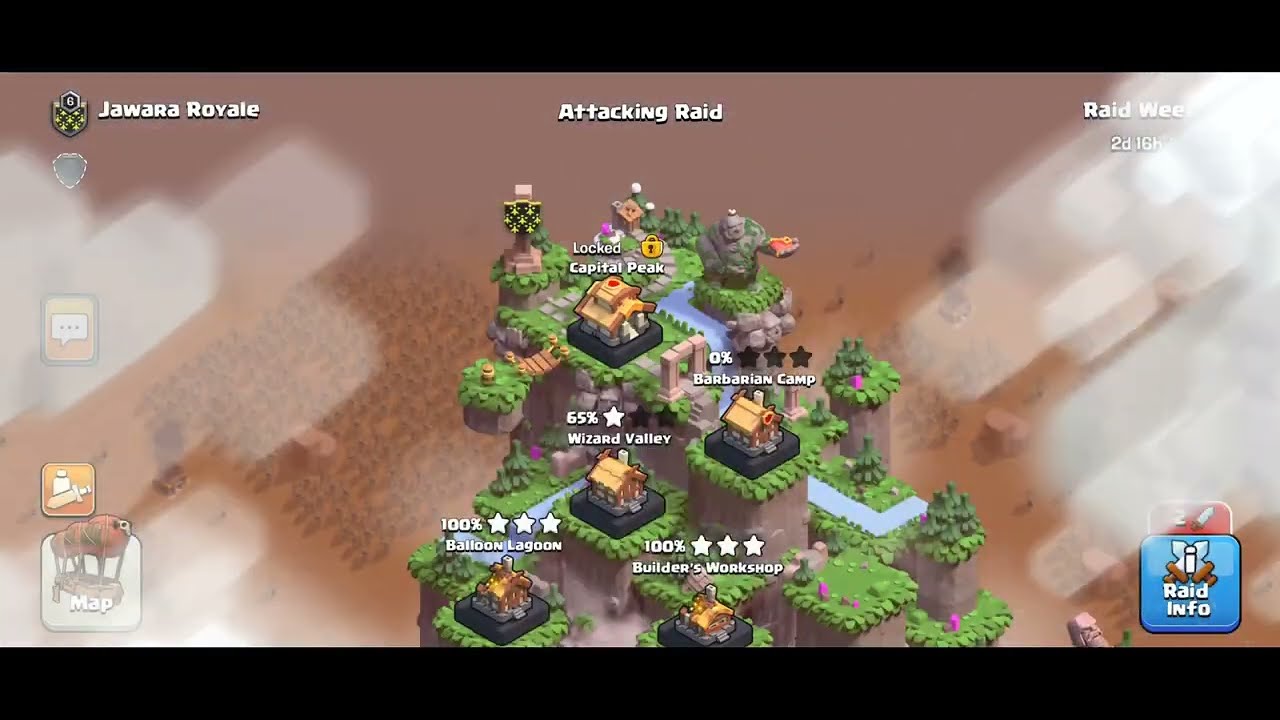The image depicts a computer screen showcasing a video game interface with a brown backdrop. At the top left corner, the text "Jawara Royale" is prominently displayed. Centered at the top, it reads "Attacking Raid," while to the right, it states "Raid Week, 21 days, 16 hours." The main animation in the center features a green tiered mountain, with each tier housing different buildings labeled with their respective statuses and completion percentages: "Locked Capital Peak," "0% Barbarian Camp," "65% Wizard Valley," "100% Balloon Lagoon," and "100% Builders Workshop." To the bottom left, there's an icon labeled "Map." The bottom right corner features a blue square with the words "Raid Info" accompanied by an icon of two swords. The scene is adorned with fine details such as white light slashes on the far left and right, adding depth to the game's interface.